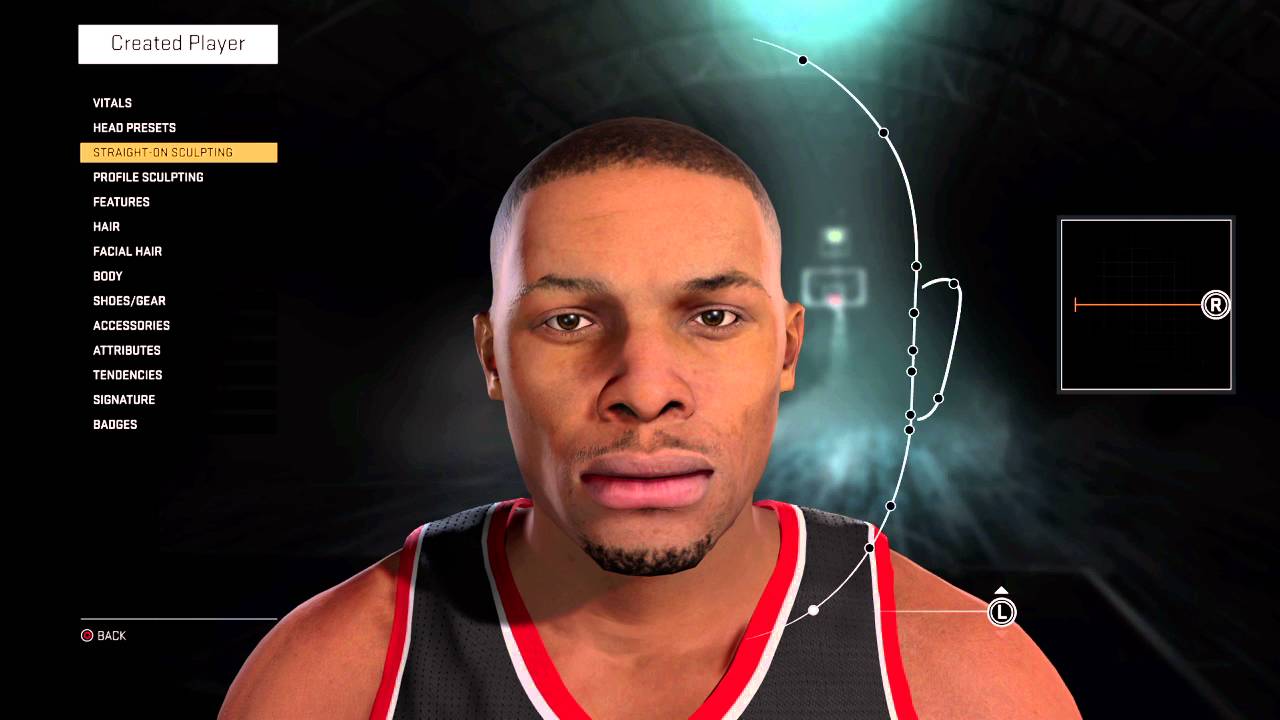Screenshot of a 3D animated basketball game displaying the "Create a Player" interface. The player being customized is a Black man with a short, fade haircut and prominent features, including big pink lips. He is attired in a striking black jersey with red and white trim. The character bears a resemblance to NBA star Giannis Antetokounmpo. The interface showcases detailed customization options, allowing users to adjust various aspects of the player's appearance and attributes. Categories listed on the left include "Vitals," "Head Presets," "Straight On Sculpting" (highlighted in yellow), "Profile Sculpting," "Features," "Hair," "Facial Hair," "Body," "Shoes/Gear," "Accessories," "Attributes," "Tendencies," "Signature," and "Badges." Navigation controls are provided for adjusting the direction of the player's head. A "Back" button is visible, indicating a return to the main menu. The interface suggests an immersive and detailed customization experience, promising an engaging gameplay.